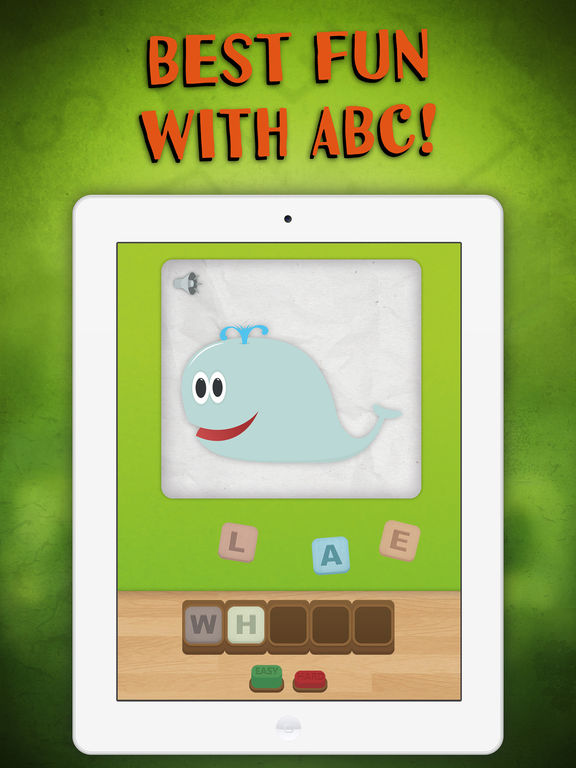The background of the image is a gradient blend of various shades of green, ranging from light green to dark green. Centered at the top, bold red text with black-bordered capital letters reads: "Best Fund with ABC!" Beneath this text, there is a rounded rectangular box with a white border. Inside this box, at the top, a black dot is centrally positioned. Below this, another smaller box with a light green background is visible, topped with a gray bar. On the left side of the gray bar, there is a speaker icon. 

The central part of this smaller box features a cheerful cartoon whale that has a smiley face and water spouting from the top of its head. Underneath the whale, three squares are aligned: a pink square with the letter "L," a light blue square with the letter "A," and another pink square with the letter "E."

At the bottom of the image, there is a wooden tabletop on which a Scrabble game is laid out, including various Scrabble pieces and a board.